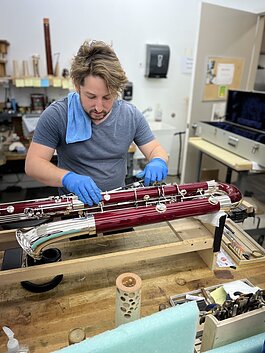In this detailed image, a man in his 30s, with short hair and a goatee, is intently working on a vintage-looking musical instrument that resembles a saxophone or another type of horn. He is seated at a wooden work table, wearing a gray t-shirt and blue gloves, with a blue rag draped over his right shoulder. The instrument is burgundy with brass and silver hardware and is held securely in place by a specialized device elevated off the table. Surrounding the man are various tools and equipment indicative of his meticulous work, stored both on the table and in a small box in front of him. Behind him, the white walls are adorned with shelves crowded with assorted items, alongside a silver instrument case that matches the one he's repairing. To the right, there's an open door with papers pinned to a board and a visible sink equipped with a black paper towel dispenser. The man’s focused expression highlights his dedication and precision in what appears to be a specialized workshop environment.